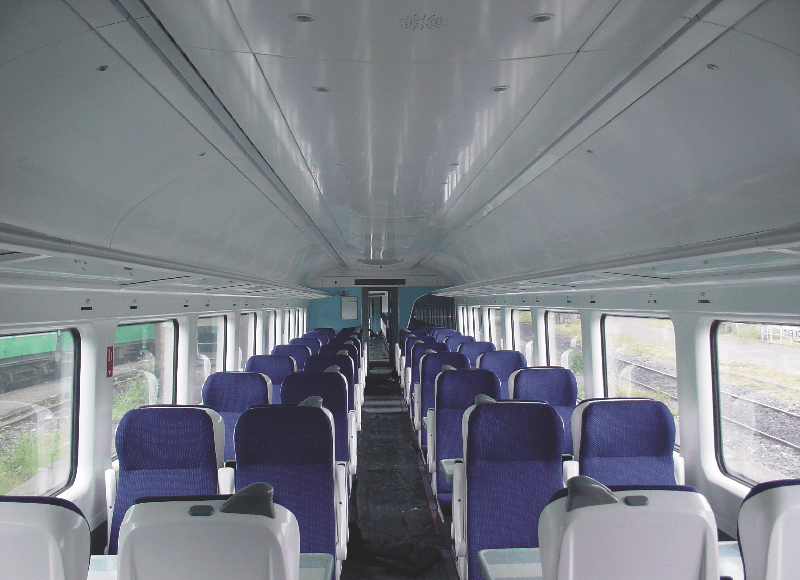The image captures the interior of a modern, empty train car, viewed from the front looking down the aisle. The train car is designed with a minimalist aesthetic, featuring white metal ceilings that curve upward, reminiscent of a school bus roof, and dark, nearly black carpeting along the aisle. The walls that divide the train cars are a light aqua or blue color. 

The seats are arranged in two rows of two on each side of the aisle, resembling the layout of a passenger jet. They have white plastic backs and are upholstered with a dark blue or bright navy fabric. The train features luggage racks running along the sides near the ceiling. 

On both sides of the car, rows of windows offer views of railroad tracks and an adjacent green train visible through the left side windows. The pristine, clean interior is accentuated by the continuity of windows that allow natural light to flood the car. The overall ambiance is serene and uncluttered, designed for functionality and comfort for its future passengers.